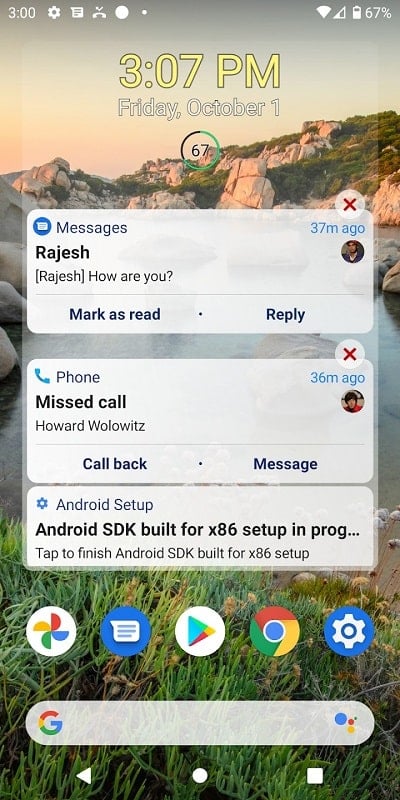The smartphone screen displays a notification interface at 3:07 p.m., as indicated by the time in yellow at the top. Below the time, it shows the date: Friday, October 1st. The status bar features various icons, including a settings gear, a speech bubble for messages, a phone receiver indicating a missed call, Wi-Fi signal strength, and a battery icon showing 67% charge within a circle that is two-thirds green and one-third black. 

The wallpaper is a serene image of a simple lake or stream, with beautiful exposed rocks and patches of green grass sprinkled throughout. The sky displays an orangish hue near the horizon, hinting at the later part of the day.

Notification details include:
- A message from Rajeesh saying, "Rajeesh, how are you?", marked as read and replied to 37 minutes ago, accompanied by Rajeesh's profile photo.
- A missed call from Howard Holowitz, with options to callback or message, recorded 36 minutes ago, also accompanied by Howard's profile photo.
- An Android setup notification indicating "Android SDK build for x86 setup in progress; tap to finish the Android SDK build."

Below the notifications, several app icons are visible, including:
- One resembling the Google pinwheel (possibly for Photos)
- A messaging icon
- The Google Play Store
- Chrome browser
- Settings icon

A Google search bar appears towards the bottom of the screen. Overlapping the grassy part of the wallpaper at the very bottom are the three navigation buttons.